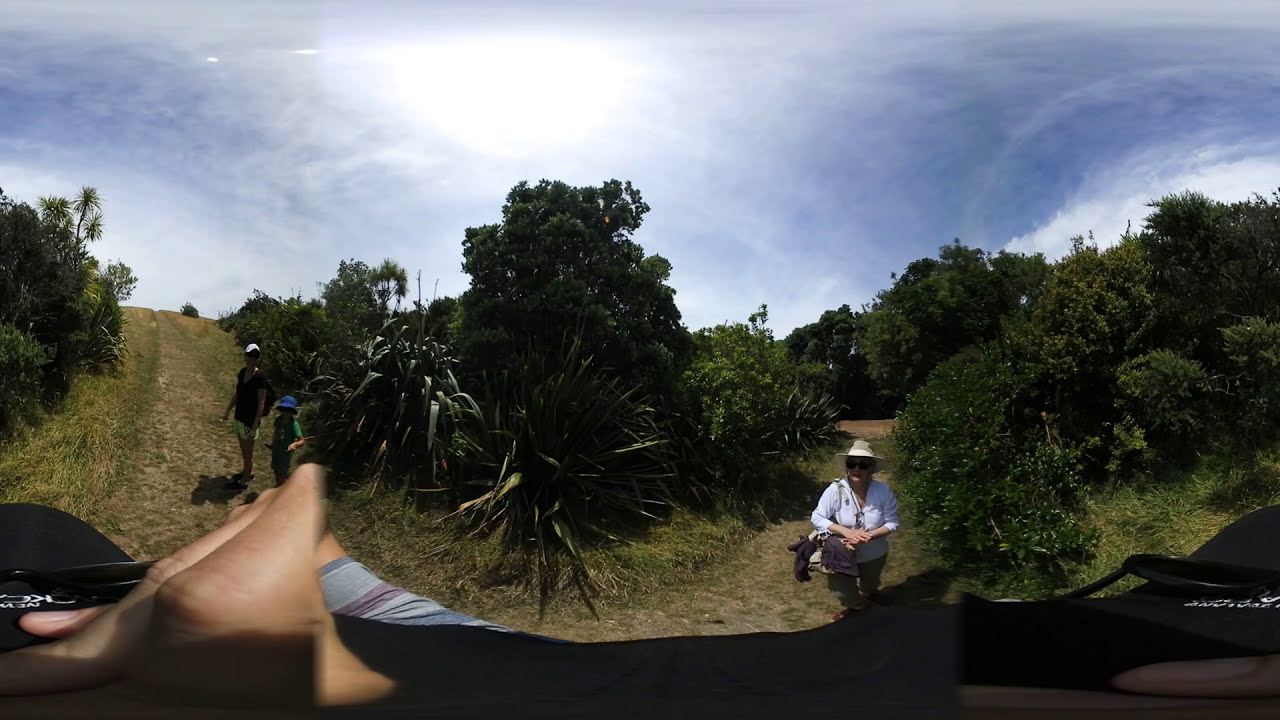The image depicts a vibrant, three-dimensional panoramic view of a lush, green landscape that appears to be a public garden or park. Central to the photograph is a well-trodden, brown trail that winds through the middle of the scene, flanked by assorted trees and manicured bushes on either side. Positioned right alongside the trail is a woman dressed in a white shirt, beige pants, and a tan sun hat, with sunglasses adorning her face and a beige bag slung over her shoulder. She appears to be fairly heavyset and has her hands crossed in front of her. To her left is an adult wearing a white cap, a black shirt, and neon shorts, accompanied by a child sporting a blue hat and a green shirt. The trail seems to rise upwards, with green grassy paths extending on both sides of the dense, tall trees. The sky above is a deep blue with sparse clouds, indicating a bright and sunny day. There is a slight suggestion of a hand or vehicle dashboard in the foreground, adding a subtle, blurred depth to the image.